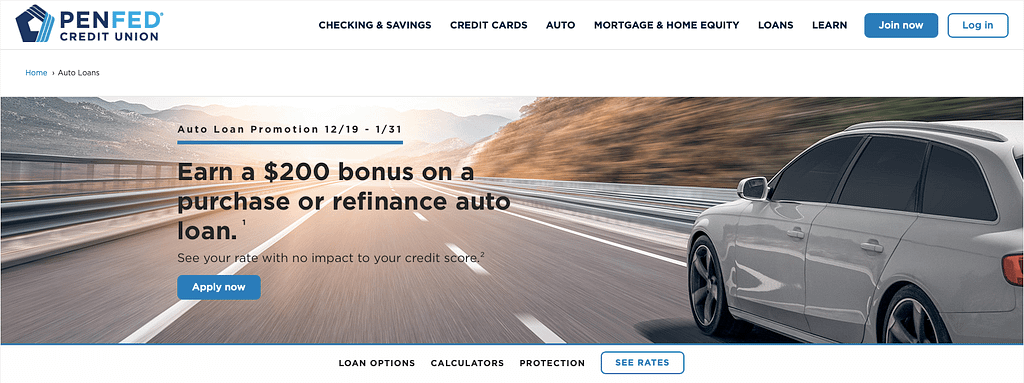This image is a computer screenshot of an advertisement for PenFed Credit Union. In the upper left corner of the image, there is a pentagon-shaped logo followed by the text "PenFed Credit Union." A black navigation bar at the top of the screen includes various sections labeled "Checking and Savings," "Credit Cards," "Auto," "Mortgage and Home Equity," "Loans," "Learn," and features a blue "Join Now" button and a white "Log In" button in the upper right corner. 

Beneath this menu, a prominent, wide rectangular photograph showcases a silver-gray SUV traveling down a road. The car is positioned on the right side of the image, moving diagonally toward the upper left. The road is mostly centered in the frame, with a dried, brown hill visible in the upper right portion, forming the background to the right side of the car and road.

Superimposed on this image is promotional text that reads, "Auto Loan Promotion 12-19-131: Earn a $200 bonus on a purchase or refinance auto loan." Below this, an "Apply Now" button is prominently displayed, inviting users to take action on the offer.